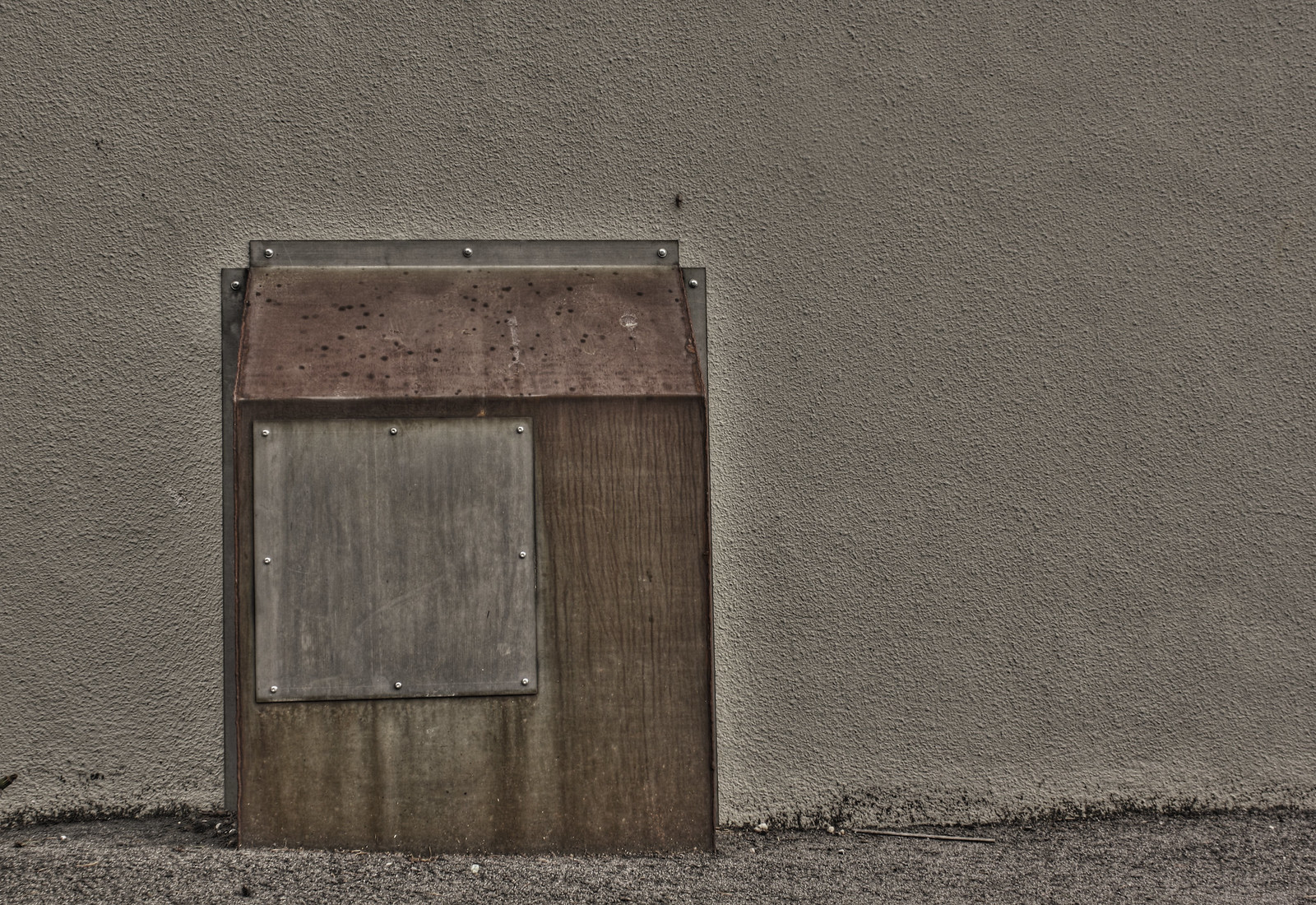The image depicts an outdoor scene featuring a textured, light gray stone wall that appears somewhat dirty with noticeable stains. Toward the left side of the wall, there is a small rectangular section that once might have served as an opening, possibly resembling a dog door that has now been sealed shut. This area is bordered by what looks like an old plastic or wooden frame, with additional wooden panels bolted over it. The upper part of this sealed section is covered in a speckled red or maroon material, which is very dirty. Below this sealed area, the ground transitioning beneath the wall appears to be a mix of fine sand, dirt, and possibly pavement, displaying an uneven surface with black spots and stains. This portion of the image suggests an outdoor shed-like structure that has been fastened securely to the wall, exhibiting many nails and a construction-like patchwork of materials, further enhancing its age-worn and utilitarian appearance.